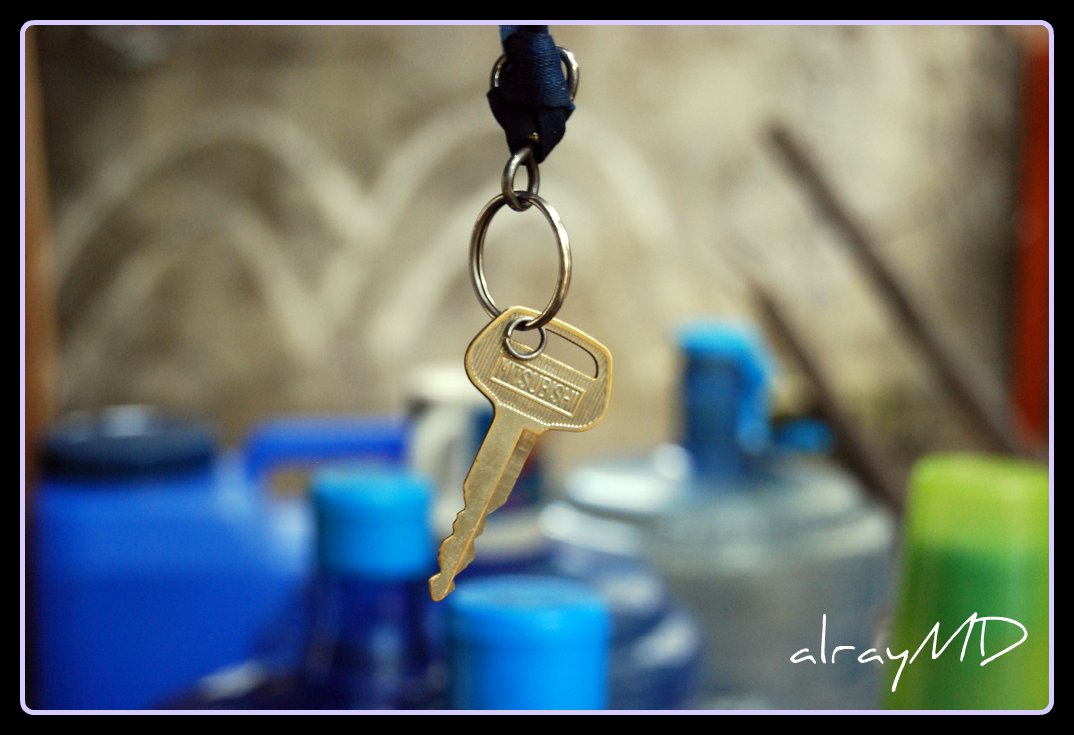The photograph showcases a bronze-colored key engraved with "Mitsubishi" hanging from a silver hourglass-shaped keyring, which is attached to a round silver keyring. This is all suspended by a blue ribbon-like keychain. In the background, a blur of various objects in whites, blues, greens, and grays adds an indistinct, colorful backdrop. Notably, the image has a watermark reading "Alray MD" in white, located at the bottom right. A tiny, partially open metal ring also dangles from the keyrings. The overall composition captures the key as the clear focal point amidst an out-of-focus, yet colorful, setting.